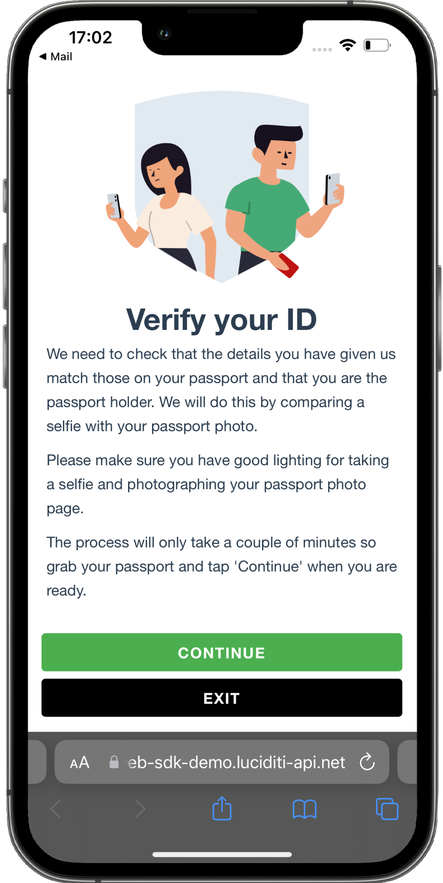The image showcases a vertically-oriented cell phone with a sleek silver edge. The device's right side features a prominent button, while the left side has three smaller protruding buttons. Framing the phone's screen is a black bezel, with a slight indent at the top housing the front-facing camera. 

Displayed on the screen, at the top amidst a white background, are the notations "1702" and "mail." The upper right corner of the display includes a Wi-Fi icon and an almost depleted battery icon, indicative of the phone's current status. Below this section, there is a cartoon depicting a man in a green shirt and a woman in a white shirt, both looking at their cell phones.

Underneath the cartoon, the screen reads: "Verify your ID. We need to check that the details you have given us match those on your passport and that you are a passport holder. We will do this by comparing a selfie with your passport photo. Please make sure that you have good lighting for taking a selfie and photographing your passport photo page. The process will only take a couple of minutes so grab your passport and tap continue when you are ready." At the bottom of the screen, there is a green "Continue" button alongside a black "Exit" button. Additional navigation options include back, forward, download, and other tab buttons.